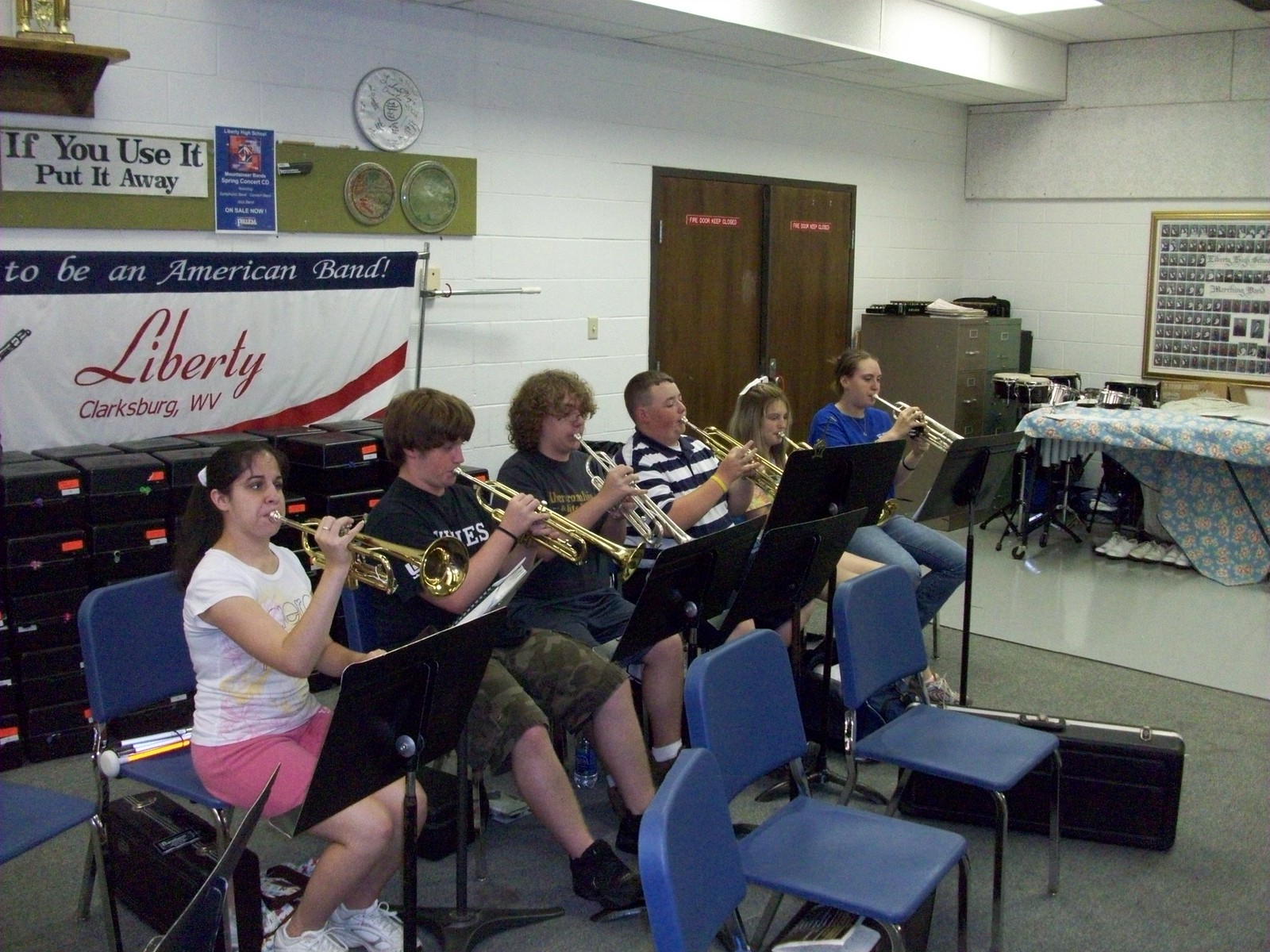This photograph captures a school band practice session in a band room, likely located in Clarksburg, West Virginia, given the Liberty Clarksburg WV banner in the background. The image is taken indoors, showing a carpeted and partially tiled floor. 

In the center of the scene, six students are seated in blue chairs, playing brass instruments, specifically trumpets. They are actively engaged, with their instruments raised to their mouths and their hands manipulating the valves. Each student has a music stand in front of them with sheet music, and instrument cases are scattered around the floor by their feet. 

The students are dressed in short sleeves, suggesting a warm climate, possibly summertime. The background reveals white-painted stone block walls adorned with clocks and signs, including one that reads "If you use it put it away." A double wooden door is also visible along the back wall. The overall color palette of the photo includes gray, black, silver, blue, pink, white, gold, and red. The room has a typical school band room setting, emphasizing the focused and organized environment of the practice session.